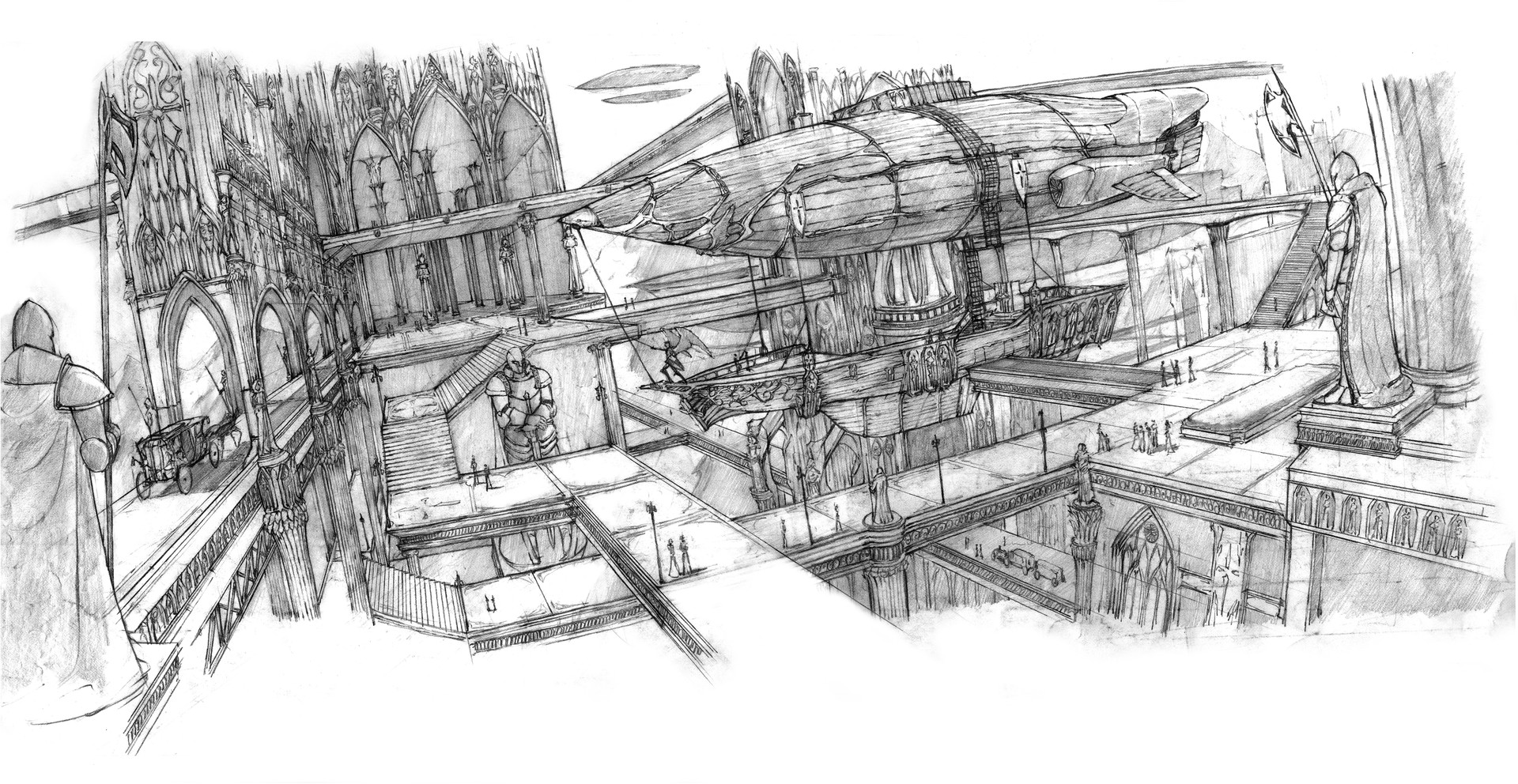This detailed and intricate black-and-white pencil sketch illustrates a bustling, fantastical world teeming with medieval and Renaissance-inspired elements. At the heart of this vivid scene is an elaborate airship, resembling a hybrid between a pirate ship and a blimp, constructed with a boat frame and sheets of wood. This airship is docked at a platform, with a person standing at the bow, sword in hand, seemingly ready for battle. Surrounding the airship are walkways and parapets reminiscent of castle architecture, with guards or knights posted strategically. The interior of the massive structure resembles a cathedral merged with an airship station, complete with vaulted entranceways and bustling passages. Dominating the left and right sides of the image are enormous statues of armored figures, framing the scene and lending an air of grandiosity. Despite the monochromatic palette, the sketch brims with activity and detail, creating a vivid tableau of a fantastical, medieval world.